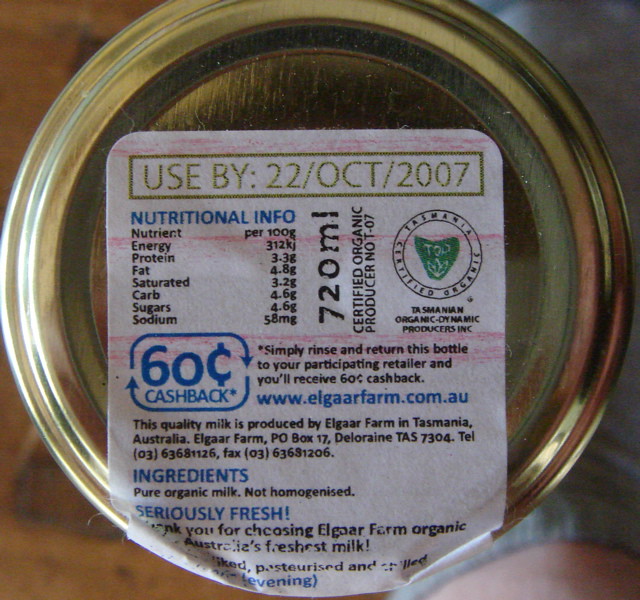### Cleaned and Detailed Caption:

A close-up bird's eye view image showcases the bottom of a bronze-colored can with a sticker label attached to it. The can is held close to the camera lens, with a hand visible behind it on the right side occupying about a third of the image. The hand appears to be resting on a t-shirt, with a portion of the cloth and skin extending out of frame at the bottom right corner. 

In the background, the photo reveals a wooden table surface visible in both the top left and bottom left corners, although it remains blurred due to the camera's focus on the can.

The sticker label on the can has a white background and contains detailed text within a green-bordered rectangle. It reads: "use by 22nd October 2007" followed by a nutritional information table. The table provides the following details per 100 grams:
- Energy: 312 kilojoules
- Protein: 3.3 grams
- Fat: 4.8 grams, of which saturated fat is 3.2 grams
- Carbohydrates: 4.6 grams, all of which are sugars
- Sodium: 58 milligrams

Beside the nutritional information, there is vertical text that reads: "720 milliliters certified organic producer NOT-07." Below this, a diagram featuring two arrows forms a square symbolizing recycling. One arrow points around the top to the side at the bottom, while the other arrow goes around the bottom pointing back towards the first arrow.

Inside the square, blue text reads "60 cents cash back" with an asterisk. The asterisk note explains: "Simply rinse and return this bottle to your participating retailer, and you will receive 60 cents cash back."